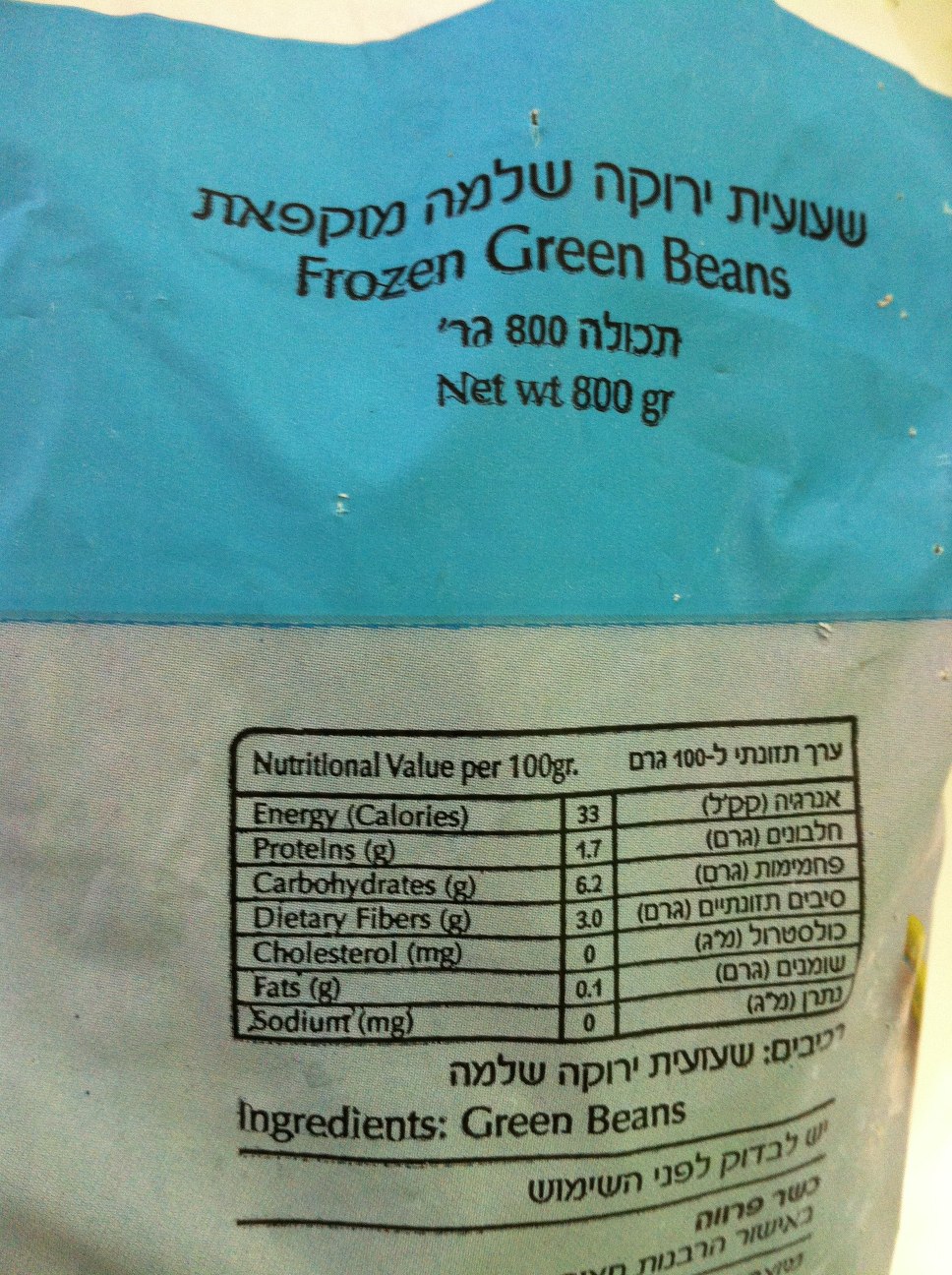This image prominently features the backside of a package of frozen green beans. The top section of the package is light blue and displays the text "Frozen Green Beans" in multiple languages. The package weighs 800 grams. The majority of the image is occupied by detailed nutritional information, which lists values per 100 grams: 33 calories, 1.7 grams of protein, 6.2 grams of carbohydrates, 3 grams of fiber, 0 grams of cholesterol, 0.1 grams of fat, and 0 grams of sodium. Below the nutritional facts, the ingredients section simply states "Green Beans." The package design is split into a blue top half and a white bottom half, where all the details are clearly displayed.